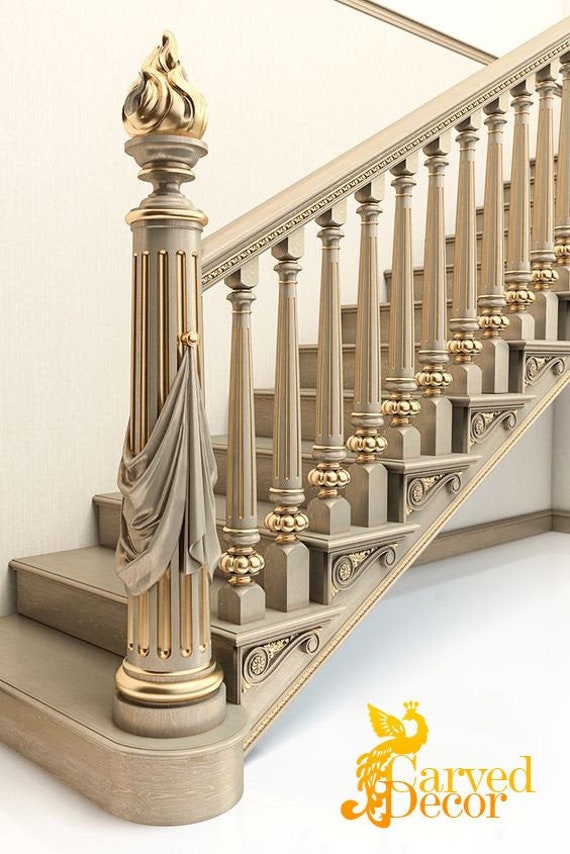This photograph captures the opulence of a Romanesque-inspired, intricately carved marble staircase with gold accents. The white marble steps, numbering around fifteen, rise majestically against a beige wall with a brown trim at the base. On the right side, each step features a gold and yellow emblem resembling a dragon or phoenix alongside ornate carvings. The staircase is adorned with an elaborately detailed banister, seemingly marble and gilded with gold highlights, particularly at the base of each railing. A grand pillar at the bottom right, crowned with an ornate cap and bright gold accents, anchors the staircase. Golden scrollwork and floral-like designs embellish the spindles and railings, while a continuous gold stripe traces the edge of the staircase, enhancing its luxurious appearance.